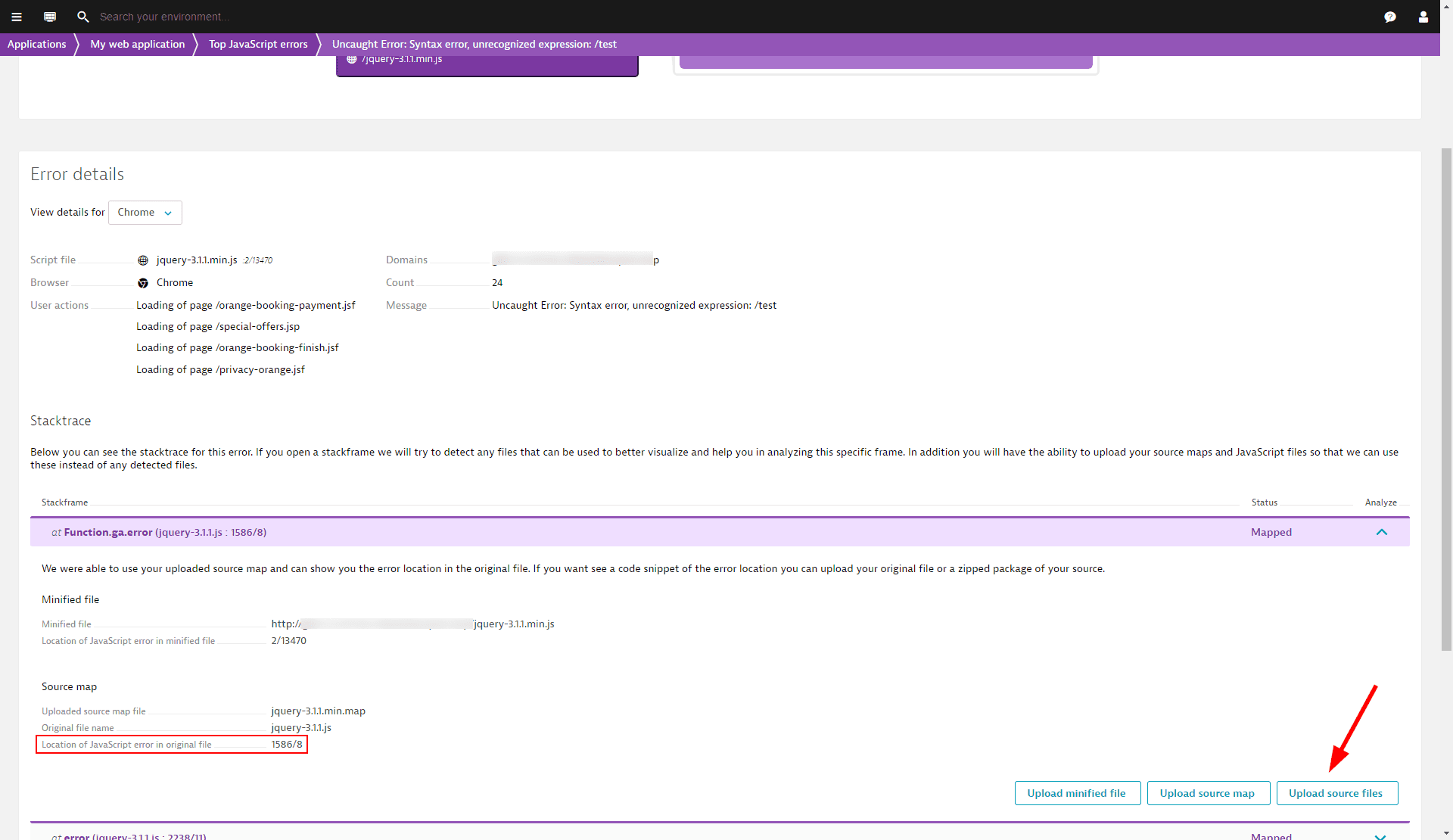**Detailed Descriptive Caption:**

The image is a screenshot of a browser-based error monitoring interface. In the upper left corner, there is a search bar featuring a white magnifying glass icon. Directly below the search bar is a green horizontal band that contains several menu options, reading from left to right: "Applications," "My Web Application," "Top JavaScript Errors," "Uncaught Error," "Syntax Error," and "Unrecognized Expression Test."

The central area of the screenshot displays a white background section that provides detailed error information. This section includes headings such as "Error Details" along with an actionable button labeled "View Details for Chrome," which features a blue arrow pointing downward. Beneath this, you can see categorized details like "Script File," "Browser," and "User Actions."

On the right side of the error details section, there is a segmented area displaying information under the headings "Domains," "Count," and "Message." It shows an entry with "24" counts of an error message reading "Uncaught Error: Syntax Error, Unrecognized Expression Test."

Finally, a prominent purple horizontal banner spans the width of the screenshot. This banner is labeled with key terms "Function," "Error," and "jQuery."